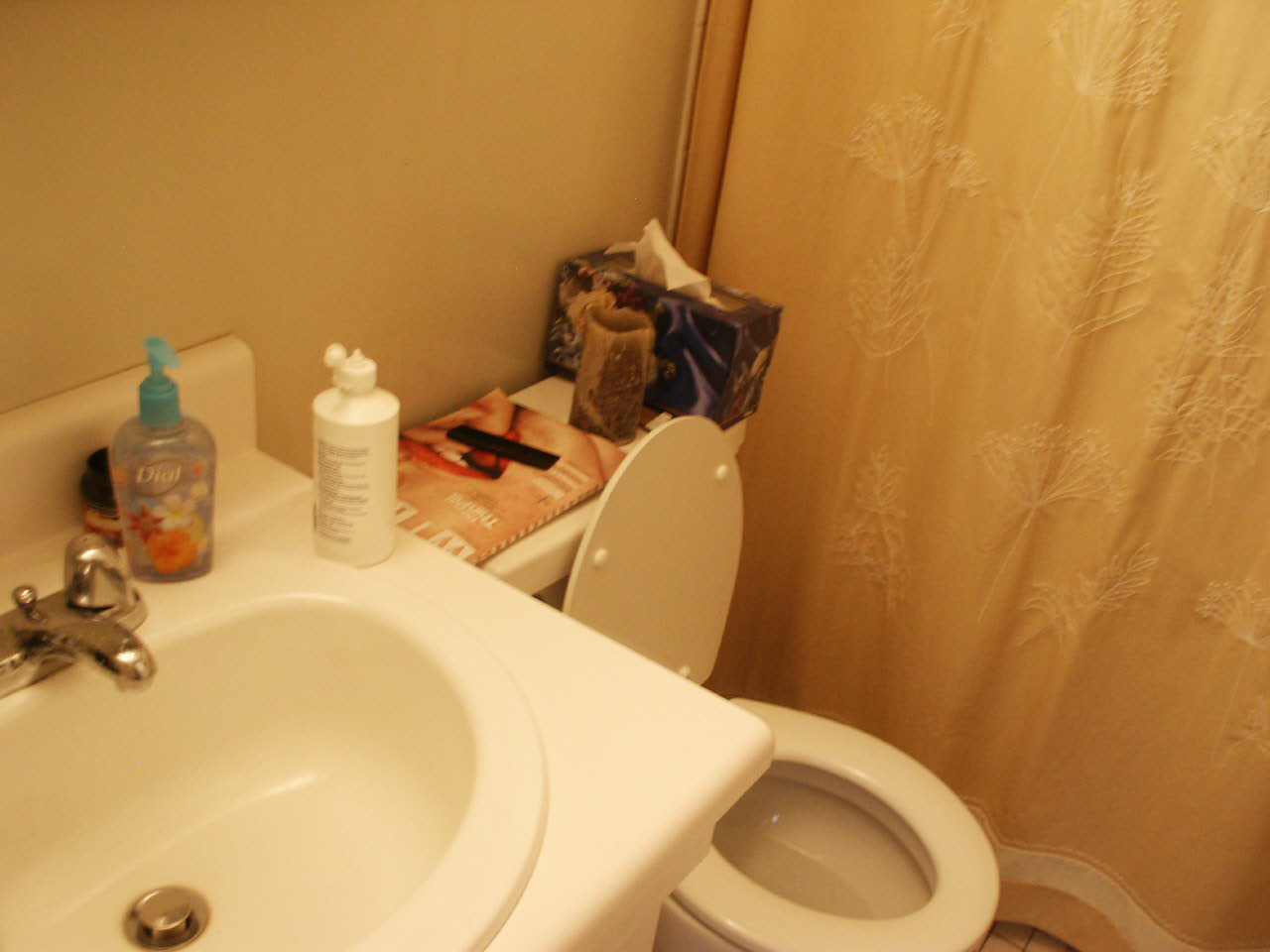This image captures a bathroom scene taken from the left side of the room, facing towards the right. On the bottom left corner of the image, reaching up towards the center-left, is part of a bathroom sink. On the sink, there is a squeezable bottle, possibly containing a saline solution for contact lenses. Next to it, there is a soap dispenser pump and an obscured object behind it. To the right of the sink, a toilet is visible with the lid up and the seat down. On top of the toilet's reservoir, there is a neatly placed magazine with a comb resting on it, alongside a candle and a box of tissues.